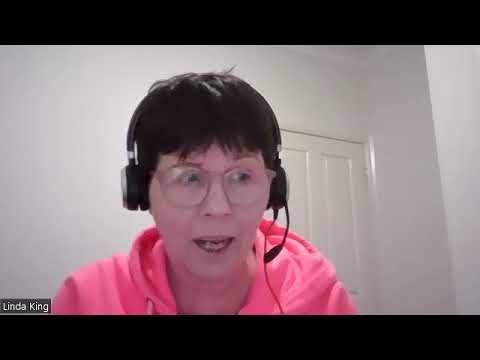The image captures a woman, Linda King, likely in her late 50s or 60s, during a Zoom call. She wears a pink sweatshirt under a black headset equipped with a microphone positioned in front of her mouth, which is slightly open as if she is speaking. Her short hair, which might be brown or black, is styled with bangs reaching her eyebrows and shorter sides. Large, possibly transparent, reading glasses frame her face. The background is a plain white wall with a closed white door on the right. The name "Linda King" is displayed in a small box at the bottom left corner, and the image has black borders at the top and bottom, indicating it might be a low-resolution screenshot. Linda appears to be engaging in conversation, looking slightly to her left.